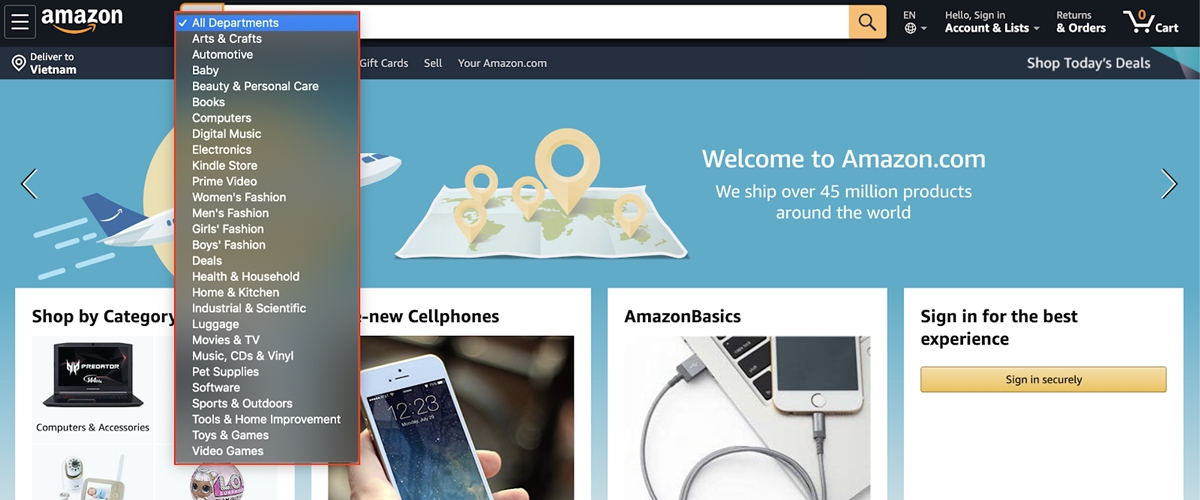This screenshot captures the Amazon homepage that includes a variety of elements presenting a structured, user-friendly interface. In the top-left corner, the Amazon logo is prominently displayed next to a menu icon consisting of three horizontal bars. Adjacent to this, the page shows the search bar centered at the top, equipped with an orange magnifying glass symbol for easy access.

The site is set to English, and the top navigation bar includes links labeled "Hello, Sign in," "Account & Lists," "Returns & Orders," and a shopping cart icon, which currently indicates zero items. Directly below the Amazon logo, there's a delivery location notice stating "Deliver to Vietnam."

The left-hand side of the page features a drop-down menu for selecting different departments, currently set to "All Departments," but allowing for an alphabetical selection of various categories. Dominating the central area, a welcoming banner reads, "Welcome to Amazon.com. We ship over 45 million products around the world," complemented by a graphic showcasing a global map adorned with location pinpoints and an airplane flying over the sun.

Below this banner, the page splits into three sections showcasing various products and categories. The left section is titled "Shop by Category," the middle section partially displays "New Cell Phones," hampered by the overlapping drop-down menu, and the right section highlights "Amazon Basics" with accompanying product images.

At the bottom-right corner of the page, a call-to-action prompts users to "Sign in for the best experience," emphasized by an orange "Sign in securely" button, reinforcing Amazon’s focus on personalized user experience.